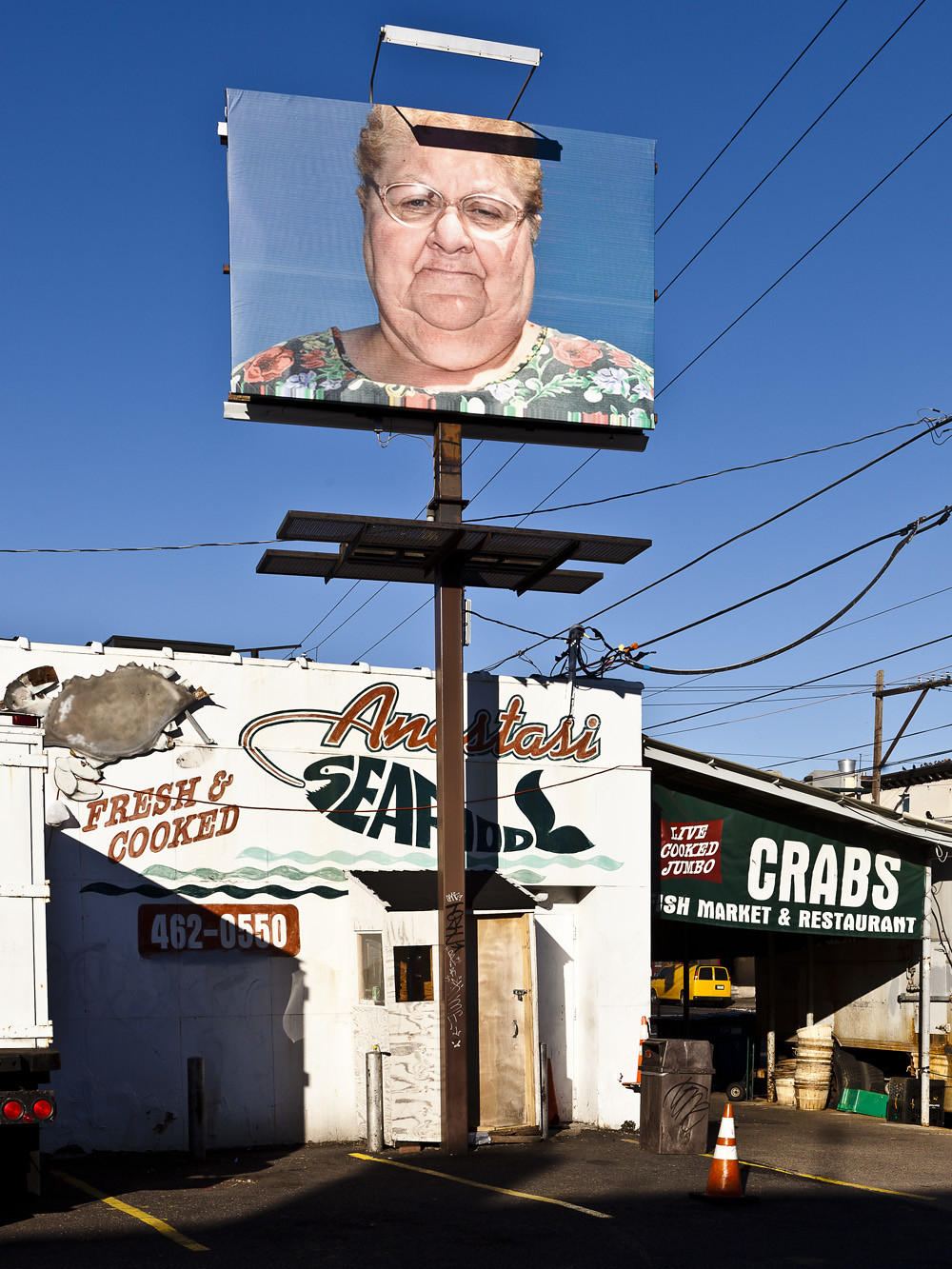In this vertically rectangular image, captured outdoors with natural lighting, the upper portion showcases a gradient blue sky, transitioning from a dark blue at the top to a lighter blue towards the center. Dominating the lower portion of the frame is the side of a building that stretches horizontally from left to right. Just to the right of the center, a canopy juts outward from the building, adorned with a black banner that reads, "Live Cooked Jumbo Crabs Fish Market and Restaurant." The building's wall features some artwork, including the phrases "Fresh and Cooked" alongside a visible phone number. In front of the wall stands a large, square brown steel post that supports a prominent billboard above. This billboard displays an image of a woman with a heavy-set face, wearing glasses and a white floral-patterned shirt, with only the top of her shoulder visible.